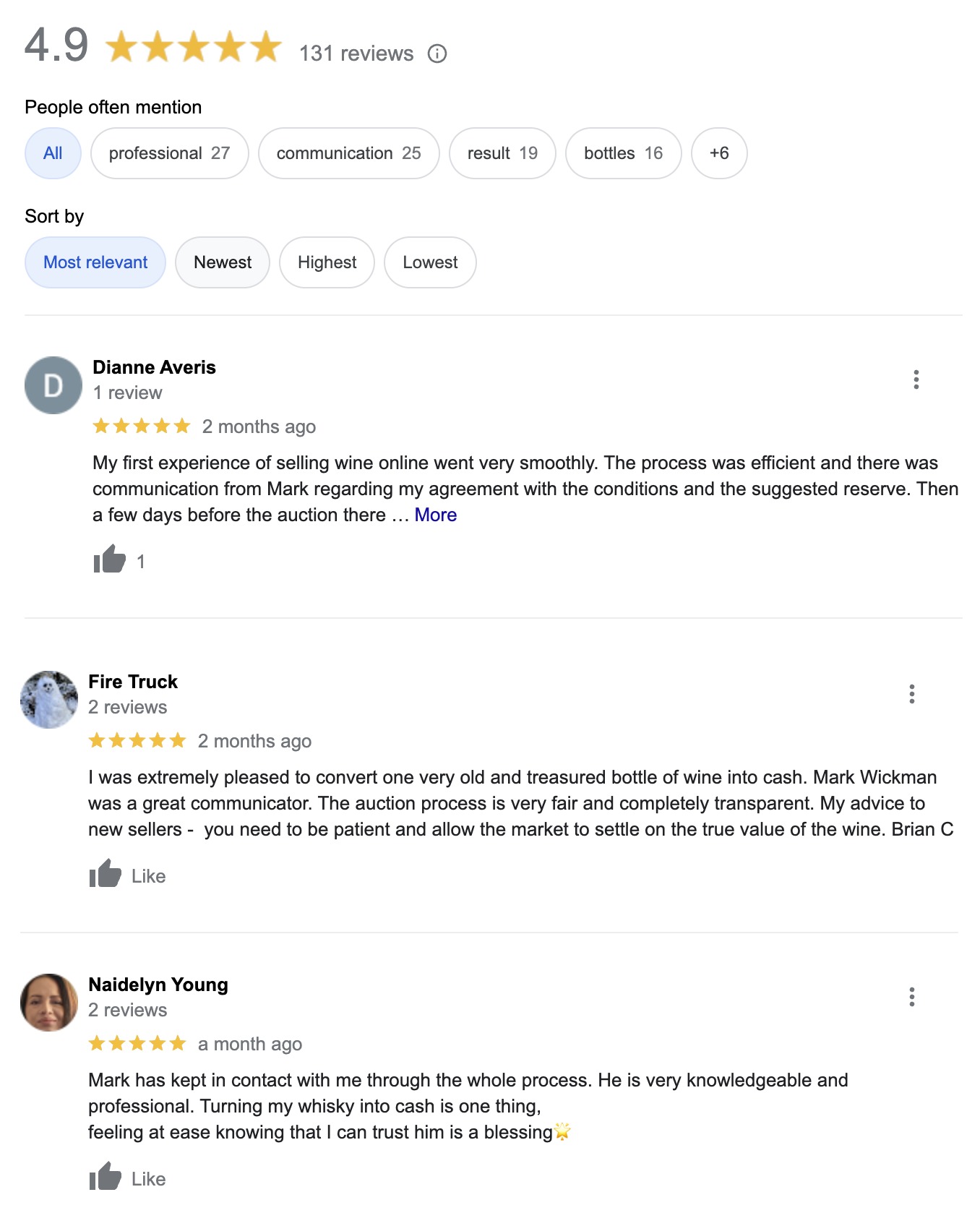This image showcases a detailed overview of reviews for a wine auction service. At the top of the image, a stellar rating of 4.9 out of 5 stars is prominently displayed alongside five stars, and it highlights that there are 131 reviews. The feedback indicates that users frequently mention the terms "professional" (27 mentions), "communication" (25 mentions), "result" (19 mentions), and "bottle" (16 mentions). Options are provided to sort the reviews by the most relevant, newest, highest, and lowest ratings.

Below this summary, three specific reviews are featured:

1. **Diane Everest**:
   - Diane shares her first-time experience selling wine online, describing the process as very smooth and efficient. Mark provided continuous communication regarding the agreement on conditions and the suggested reserve price. A few days before the auction, additional updates were given, contributing to a positive experience. Diane's review received a "thumbs up" from the community.

2. **Fire Truck**:
   - Fire Truck expresses immense satisfaction in converting an old and valuable bottle of wine into cash. They commend Mark Wickman for his excellent communication skills, praising the auction process for being fair and transparent. Fire Truck advises new sellers to exercise patience to allow the market to determine the genuine value of their wine.

3. **Natalyn Young**:
   - Natalyn appreciates the consistent contact Mark maintained throughout the entire process. She acknowledges his expertise and professionalism, highlighting the importance of trust in turning whiskey into cash. For Natalyn, feeling at ease with Mark's handling of the transaction was a noteworthy benefit.

These reviews collectively paint a positive picture of the service, emphasizing effective communication, professionalism, and customer satisfaction.